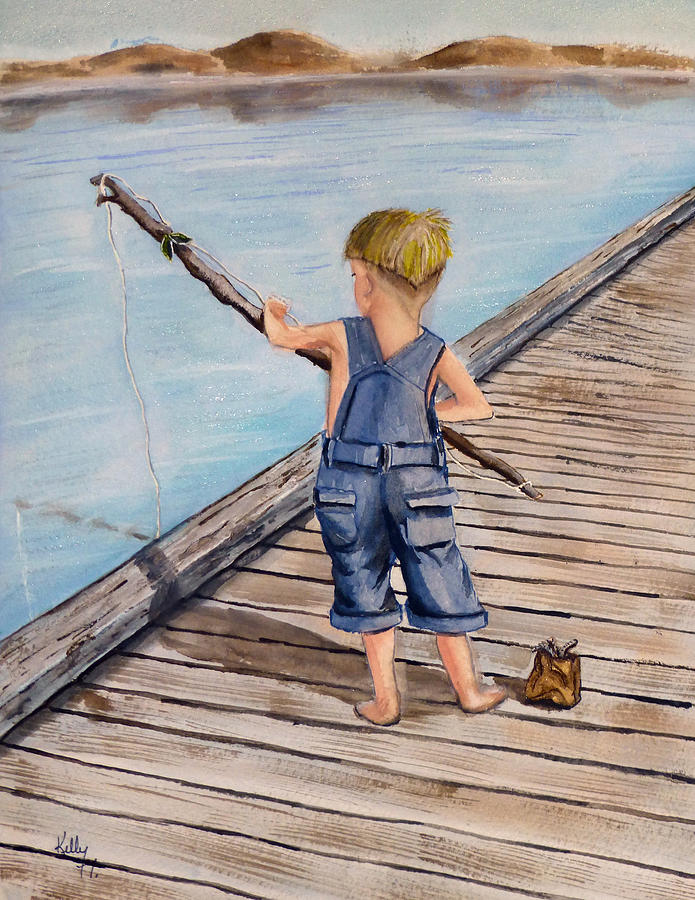In this detailed painting, a young boy with short reddish hair stands barefoot on a diagonally-stretched wooden pier, wearing only blue denim overalls. With his back to us, he stabilizes a makeshift fishing rod—a simple stick with a thick white string—over the edge of the dock, dipping it into the water below. Resting at his feet on his right side is a brown paper bag, brimming with worms. The tranquil scene captures the boy's intent focus on fishing, with the soft ripples of the water reflecting both the stick and string. In the background, serene orange hills rise above the horizon, their reflection faintly mirrored in the water's surface. The image, signed by the artist Kelly in the bottom left corner, completes the rustic and peaceful depiction.